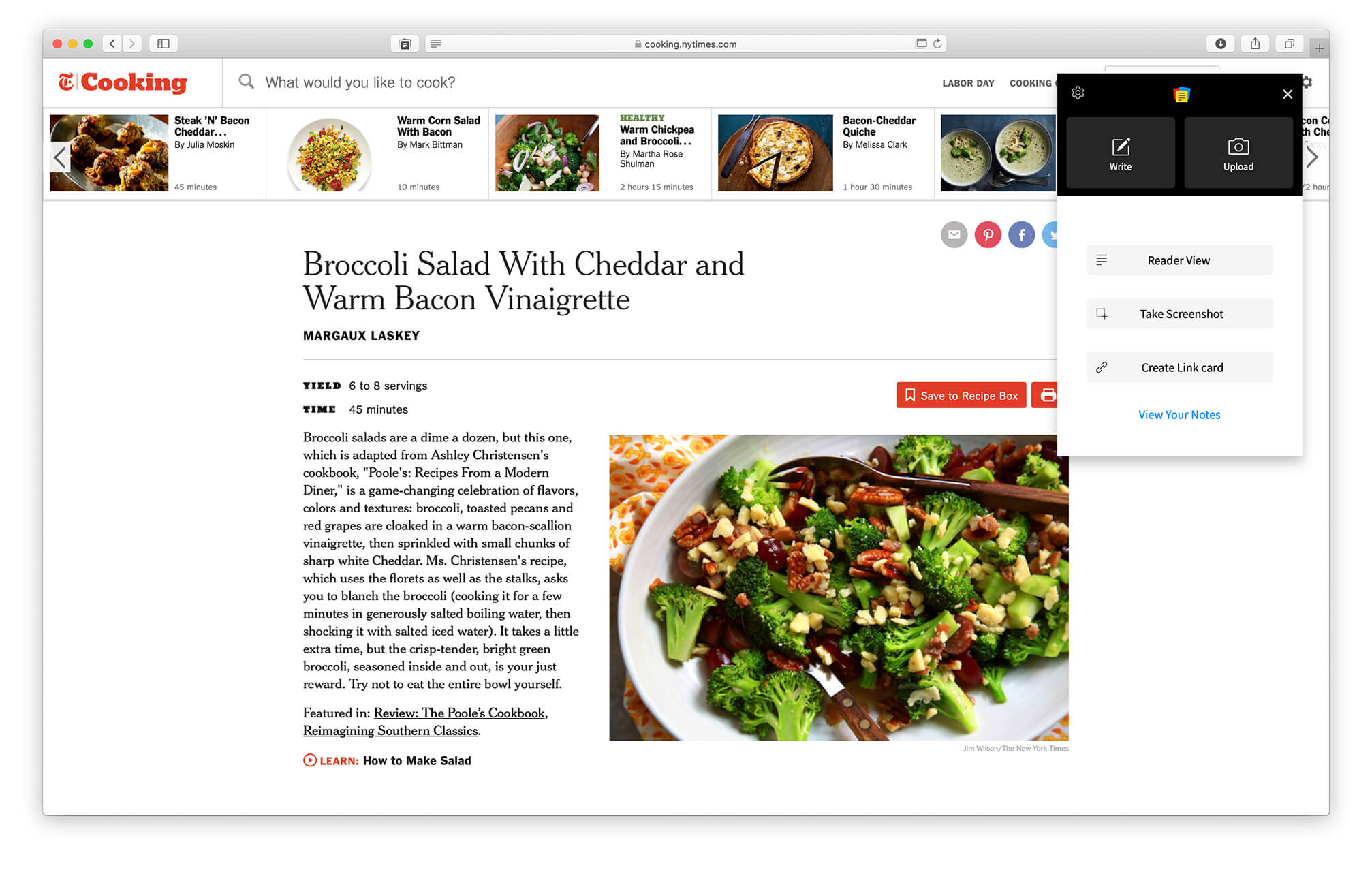The screenshot captures the New York Times cooking page in landscape mode. In the upper right-hand corner, there's a prominent pop-up box. The top section of this box has a black background. On the upper left of this section, there's a settings icon. In the center, there's an icon featuring red, blue, and yellow colors. On the upper right of the pop-up box, there's an 'X' button to close it. 

Just below the top section, the next row features two buttons labeled "Write" and "Upload". Underneath this, there's a larger white section with three slightly off-white buttons labeled "Reader View," "Take Screenshot," and "Create Link Card." Below these buttons, there's a light blue link with the label "View Your Notes," indicating a live link.

The main section of the screenshot highlights a recipe from the New York Times titled "Broccoli Salad with Cheddar and Warm Bacon Vinaigrette" by Margot Lasky. The recipe yields six to eight servings and takes approximately 45 minutes to prepare. A detailed description of the recipe is provided.

At the bottom of the page, there's a small link labeled "Learn How to Make Salad," which appears to be a video tutorial. Above the image of the Broccoli Salad with Cheddar and Warm Bacon Vinaigrette, there are two red buttons: one for "Save to Recipe Box" and another for "Print".